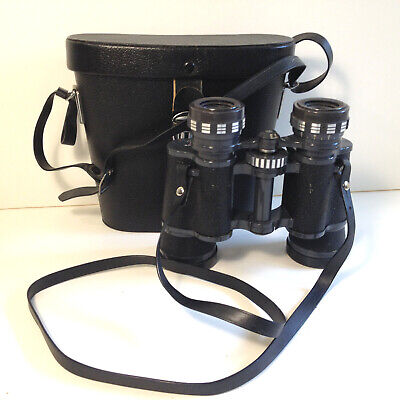The image features an old pair of black binoculars with a textured, sandpapery surface where you hold them, indicating signs of aging with some scratches. The binoculars have two eyepieces, front lenses, and adjustment dials with silver and black lining both in the center and around the eyepieces. They come with a long, black leather strap. Located behind the binoculars is a hard black leather case with a lid, resembling a basket, also equipped with a strap. The setup is displayed on a white background, likely intended for an online listing, and the entire composition has a warm yellowish tint, possibly due to lighting conditions.